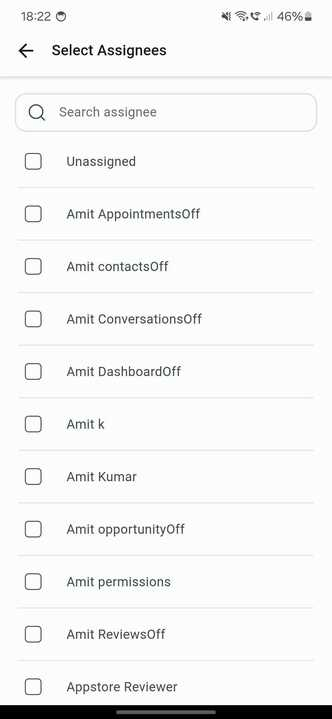This image is a detailed screenshot taken from a phone, presented in portrait orientation and significantly taller than it is wide, likely by a factor of two or three. The image is set against a grayish-white background with grayish-black font.

At the very top, the time shows as 18:22 (6:22 PM) with a circular icon next to it, which is unfamiliar. To the right of this, there are several icons: a phone controlled by remote icon, a fully filled Wi-Fi signal meter, a phone with a Wi-Fi signal emitting from it, and a network status bar displaying one out of three bars. Additionally, a vertical battery icon shows 46% charge, with the battery meter filled in black.

Beneath this status bar, a left-facing arrow points to the left, followed by a black header with the text "Select Assignees," separated by a thin horizontal gray line. Below this header, there is a light gray text box with a magnifying glass icon, labeled "Search Assignee."

The main content area consists of multiple equally sized results, separated by thin gray horizontal borders. Each result features text on the right and a checkbox on the left. The options listed are:
- Unassigned
- Emmet Appointments Off
- Emmet Contacts Off
- Emmet Conversations Off
- Emmet Dashboard Off
- Emmet K
- Emmet Kumar
- Emmet Opportunity Off
- Emmet Permissions
- Emmet Reviews
- App Store Reviewer

At the very bottom, a thin horizontal black bar spans the entire width. None of the checkboxes next to these options are marked.